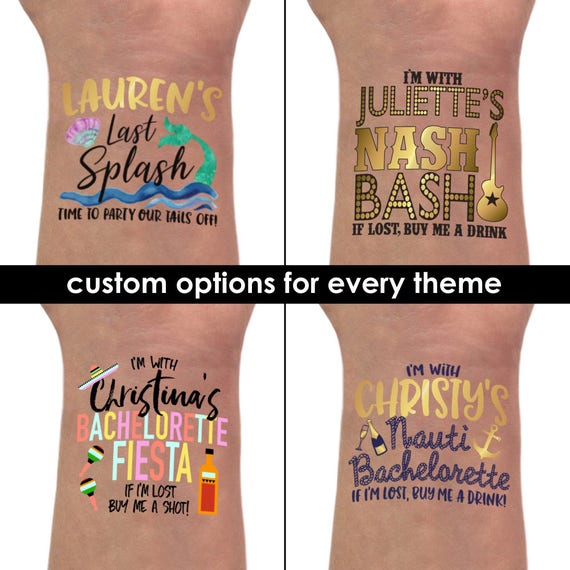The photograph features an arrangement of four inner wrist temporary tattoos, each representing a different custom event theme. The image is divided into four sections by a prominent horizontal black banner with the white text "Custom options for everything," and a thin vertical black line. 

- **Upper Left Section:** Depicts a tattoo with the text "Lauren’s Last Splash," where "Lauren’s" is in gold and "Last Splash" in black. Below, it reads, "Time to party our tails off," suggesting a mermaid-themed celebration.
- **Upper Right Section:** Showcases a tattoo with "I’m with" in black, and "Juliet’s Nash Bash" in gold. Beneath it states, "If lost, buy me a drink," also in black.
- **Lower Left Section:** Features a tattoo that reads "I’m with Christina’s Bachelorette Fiesta" in varying pastel colors and black. The phrase "If I’m lost, buy me a shot" is written in smaller black font below.
- **Lower Right Section:** Displays a tattoo which says "I’m with" in black and "Christie’s" in large gold letters. Under this, "Naughty Bachelorette" is written in black, followed by "If I’m lost, buy me a drink" in smaller letters.

This ensemble emphasizes the customizable nature of temporary tattoos for various events, each festively tailored with distinct colors and playful messages to suit bachelorette parties and similar celebrations.